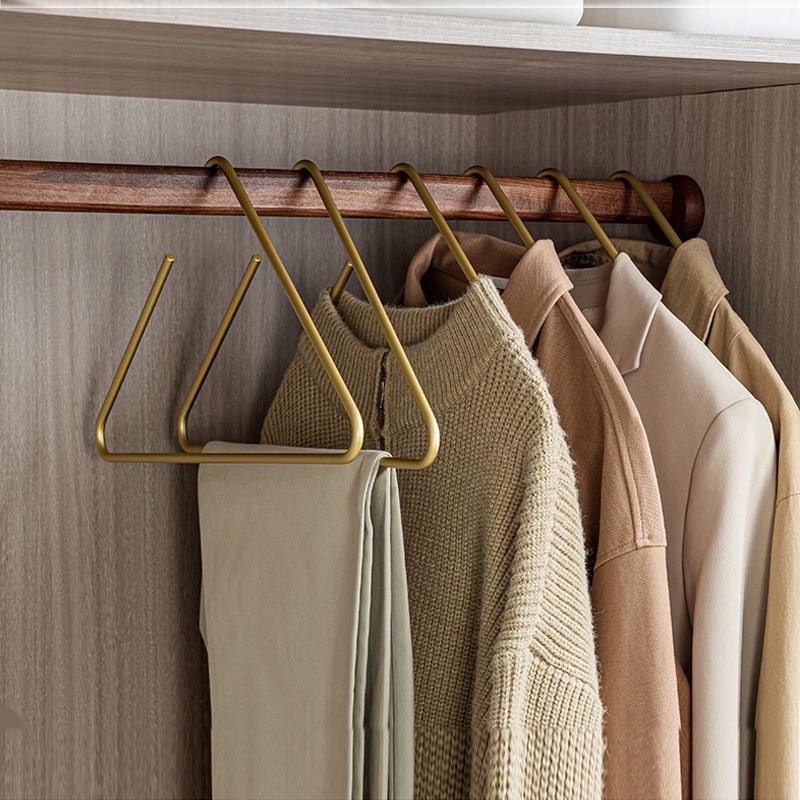The image is a square photograph showcasing the interior of a wooden closet shelf. The shelf features vertical wood grains and medium brown tones with slightly darker brown streaks, complemented by a pristine white wall in the background. The shelf is lined with several triangular gold hangers suspended from a brown beam. The first hanger, positioned on the left, is empty. Next to it, the second hanger holds a pair of neatly folded khaki dress slacks. Moving further right, the third hanger supports a light brown sweater, while the fourth holds a tan-colored jacket. The fifth hanger displays a beige jacket, followed by the last hanger, which carries a gold-colored jacket. The arrangement highlights a total of four or five garments, each meticulously hung on elegant, triangular gold hangers, illustrating a well-organized closet space.